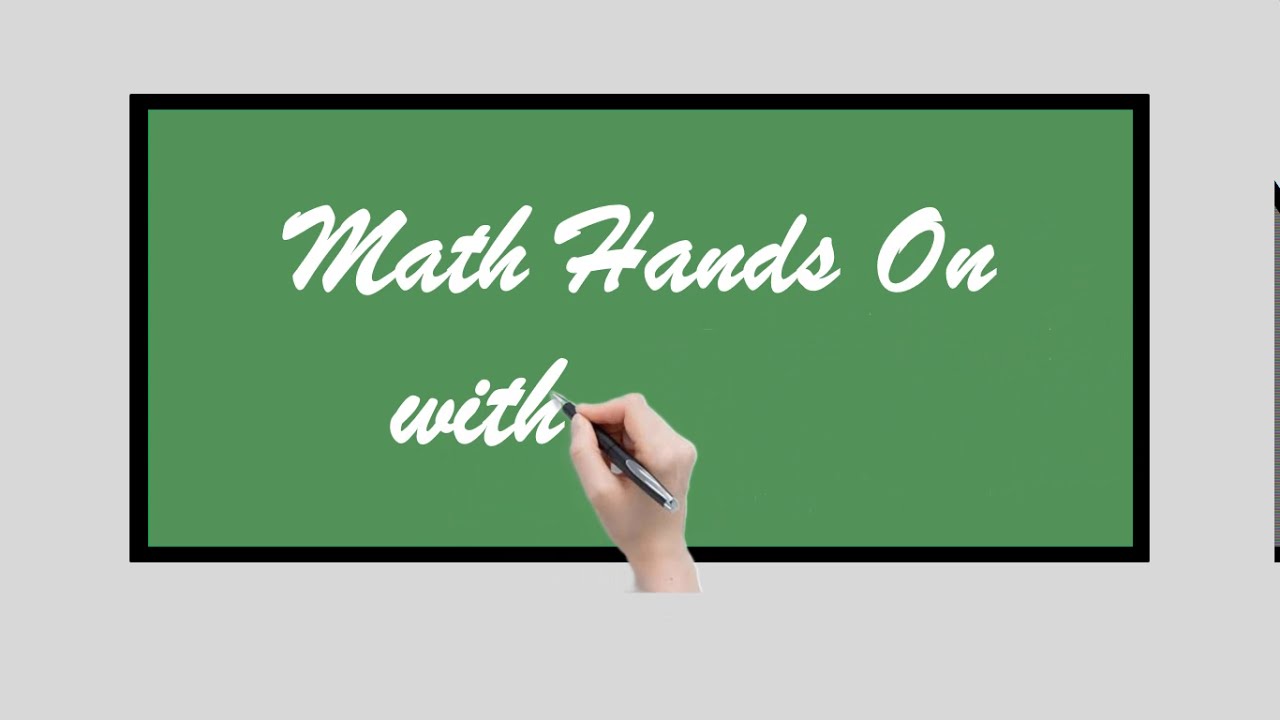The image is a screen capture from what appears to be an instructional or tutorial video. The main subject of the image is a large, horizontally oriented rectangle with a white background and a thin black border, designed to resemble a chalkboard. Inside this rectangle is a muted green area meant to mimic the traditional color of a chalkboard. A disembodied hand holding a black marker is seen hovering over this chalkboard-like area, as if in the act of writing. The text, partially written in a simple, computer-generated cursive font that appears to be chalk-like, reads "math hands-on with…". The text is in white, contrasting with the green background. The hand itself appears to be a cutout, and is notably using a pen rather than chalk, adding a modern twist to the visual. To the right of the main graphic, there is a small sliver that seems to be a continuation of another image, possibly a cropping error. The overall dimensions of the image are approximately 7 inches wide by 5 inches tall, maintaining a clear and functional design suitable for its educational purpose.